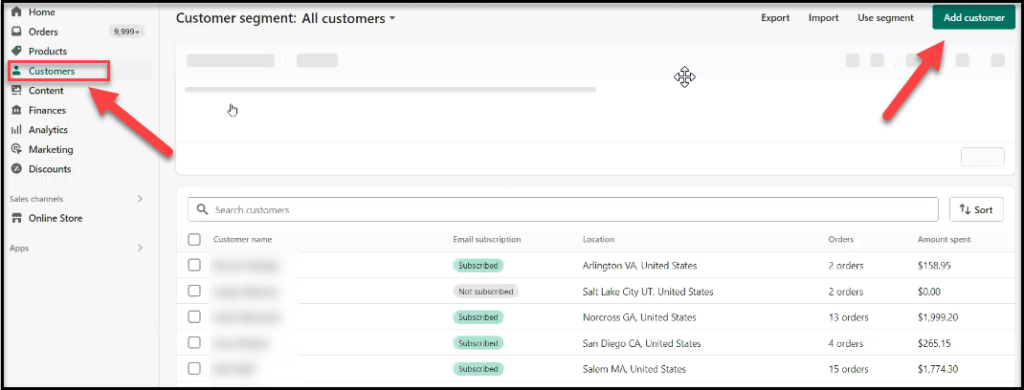This screenshot captures the "All Customers" section of an application interface, specifically focusing on customer segmentation. The layout features a vertical navigation bar on the left-hand side with options for Home, Orders, Products, Customers, Content, Finances, Analytics, Marketing, Discounts, and Online Store. Each option is accompanied by a distinctive icon, with the "Customers" section highlighted by a red outline box and indicated by a red overlay arrow.

In the upper right-hand corner, several functional buttons are displayed: "Export," "Import," and "Use Segment" in black text on a gray background. These are followed by a prominent green "Add Customer" button with white text, which is also marked by a red arrow for emphasis.

The main body of the screen features a clean, white background with gray accents, highlighting a comprehensive list of customers. To the left of each row is a checkbox for selecting individual customer entries. Currently, five customer entries are visible; however, the names are blurred out for privacy. This tabular display includes columns for Email Subscription, Location, Orders, and Amount Spent:
- **Email Subscription**: For indicating whether the customer is subscribed.
- **Location**: Showing the customer's general city and state.
- **Orders**: Displaying the number of orders placed by the customer.
- **Amount Spent**: Presenting the total amount of money the customer has spent.

This detailed layout provides an organized and user-friendly interface for managing customer information within the application.